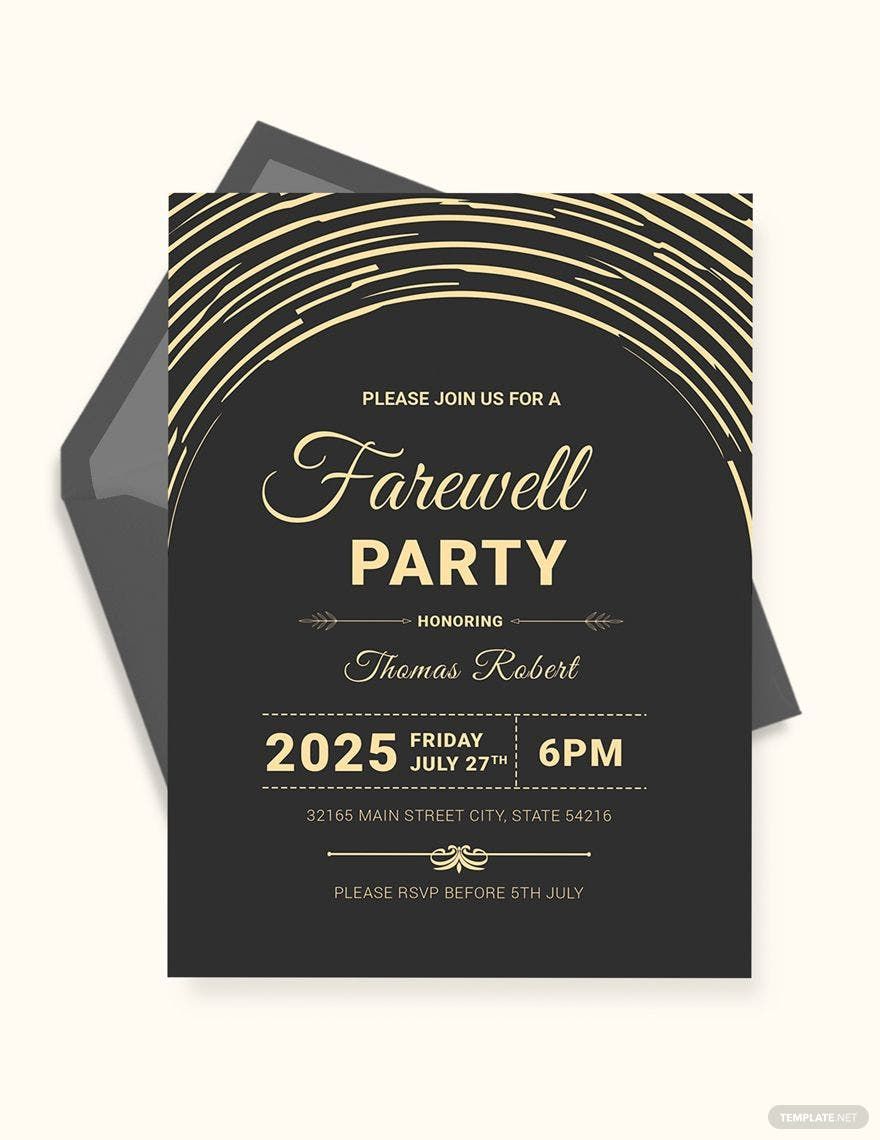The invitation showcased in the image is for a farewell party. The background of the image is a cream or beige color, with a dark charcoal or black envelope in the foreground. The invitation itself sits atop the envelope and has a predominantly black background adorned with gold or light yellow writing. At the top of the invitation, there are decorative gold-like lines forming a half-circle. The text on the invitation reads, "Please join us for a farewell party honoring Thomas Robert, Friday, July 27th, 2025, at 6 p.m.," followed by the address "32165 Main Street, City, State, 54216." It also instructs, "Please RSVP before the 5th of July," with a small decorative line above this message. The invitation combines a minimalist color scheme of black and gold/light yellow, emphasizing elegance and clarity.